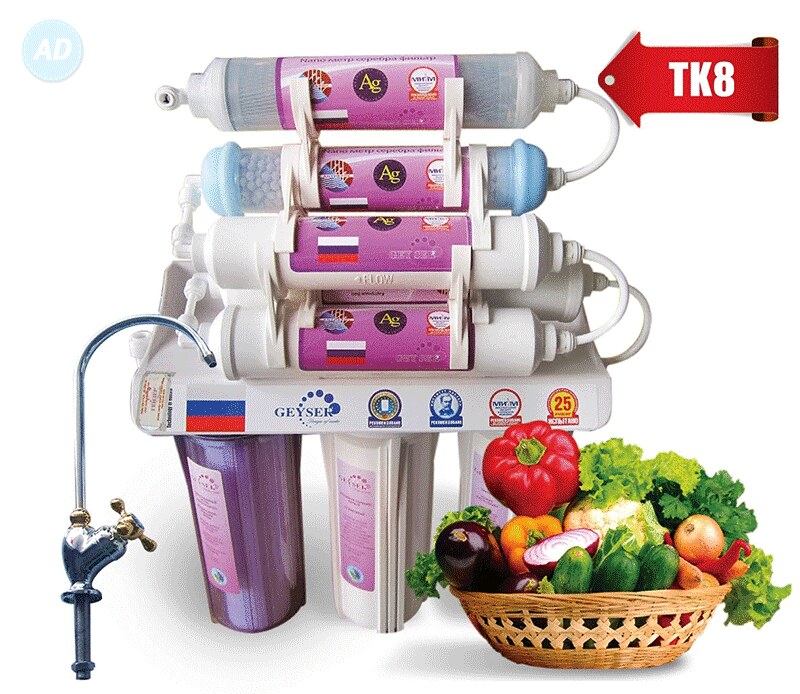The image showcases a white and purple water filtration system branded "Geischer" situated beside an array of fresh vegetables in a wicker basket. In the top left, a pale blue circle with white text says "AD". To the right, a large red arrow, labeled "TK-8" in white text, points leftward, the arrow appearing dynamic as if it can extend further. The filtration system itself features four cylindrical filters labeled "AG," arranged on a base with "Geischer" imprinted on the side. Various colored lines (white, blue, red) are visible on the left side, and the cylinders rest on a tray decorated with pink and purple stickers, presumably quality certifications. Below these, three bottles transition in color from dark lilac to white, also branded with "Geischer". An unattached, vintage-style faucet with three prongs sits to the left of the system. On the bottom right, a woven basket brims with vibrantly colored vegetables including bell peppers, eggplants, onions, kale, cucumbers, and possibly cauliflower, casting distinct shadows, implying a direct light source.